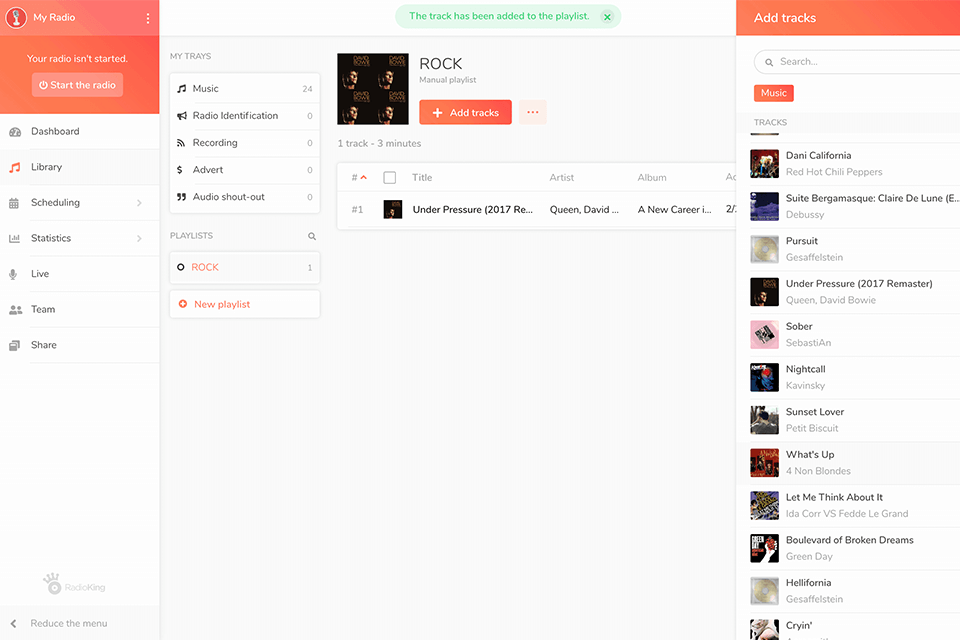The image presents a clean user interface against a white backdrop. In the top left corner, there's a paint box icon labeled "My Radio," accompanied by a vertical ellipsis on its right. Beneath this header, a notification reads, "Your Radio Is Started." A prominent pink button labeled "Start the Radio" is positioned below the notification. 

To the left, a vertical navigation panel lists various sections: "Dashboard," "Library," "Scheduling," "Statistics," "Live," "Team," and "Share." Adjacent to this, another column categorizes content under "My Trays," including entries such as "Music 24," "Radio Identification," "Recording 0," "Advert 0," and "Audio Shoutout 0."

Towards the bottom of the interface, a "Playlist" section showcases "Rock 1," and an option for "New Playlist." Next to this, the word "Rock" is displayed. Under this section is a black square featuring a nondescript image, beside which is a red rectangular button labeled "Add Tracks." Below this button, text indicates "Under Pressure 2017" by Queen and David, along with "A New Career."